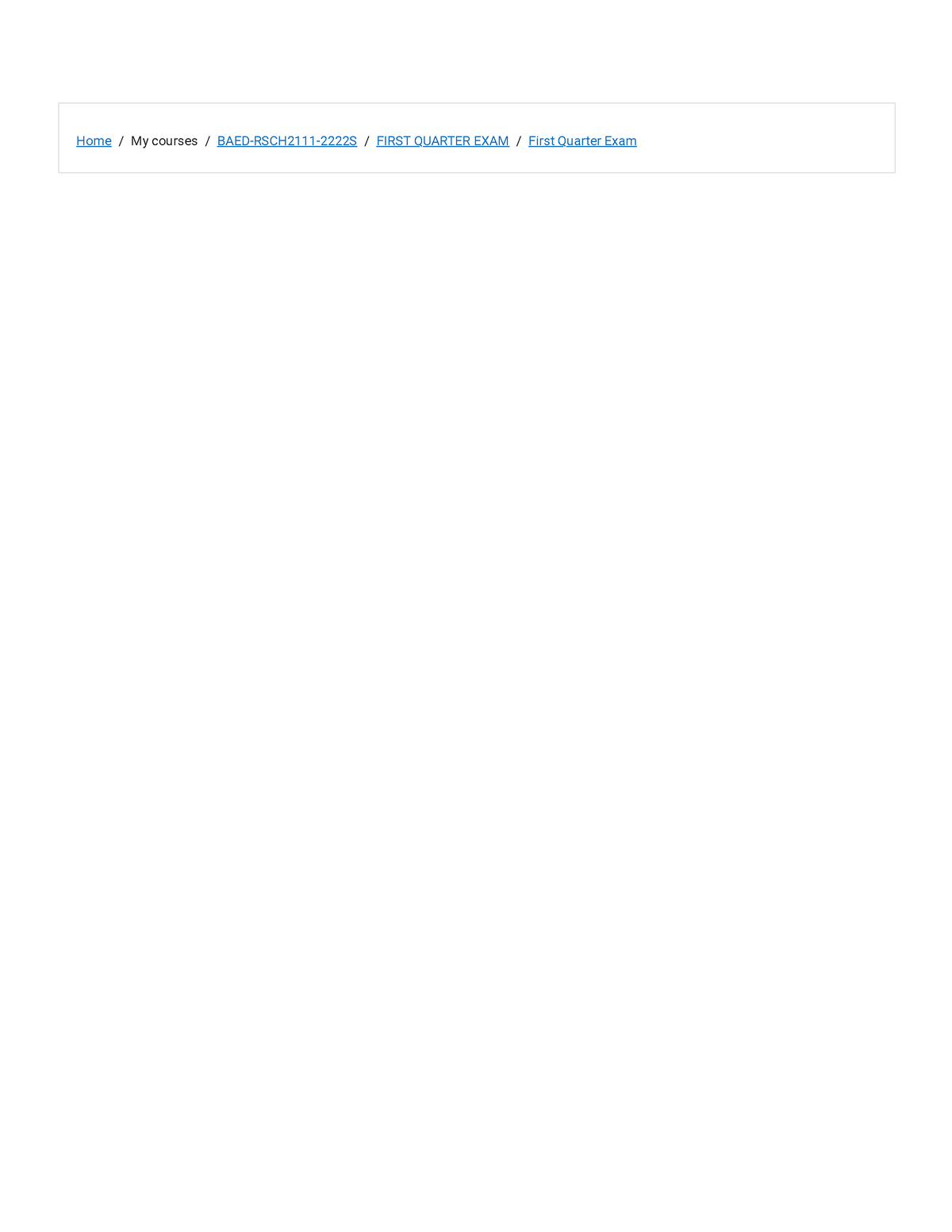The image displays a website interface, prominently featuring a navigation breadcrumb trail within a horizontal, light gray banner that stretches across the width of the page. The breadcrumb is organized as follows:

- The first item, labeled "Home," appears in blue underlined text, indicating a hyperlink.
- Following this is a separator composed of a space, a slash, and another space.
- The next item is "My Courses" in black text with a capitalized 'M.'
- Another separator (space, slash, space) follows.
- Next, there is an item labeled "BAED-RSCH2111-2222S" in capitalized blue underlined text.
- Another standard separator follows.
- The subsequent item, "First Quarter Exam," is also in capitalized blue underlined text, with spaces between "First," "Quarter," and "Exam."
- Finally, there is the label "First Quarter Exam," which is underlined with capitalized first letters for each word (i.e., "F," "Q," and "E").

Beneath this banner, the screen remains blank, indicating that no further content is displayed in the visible portion of the image.